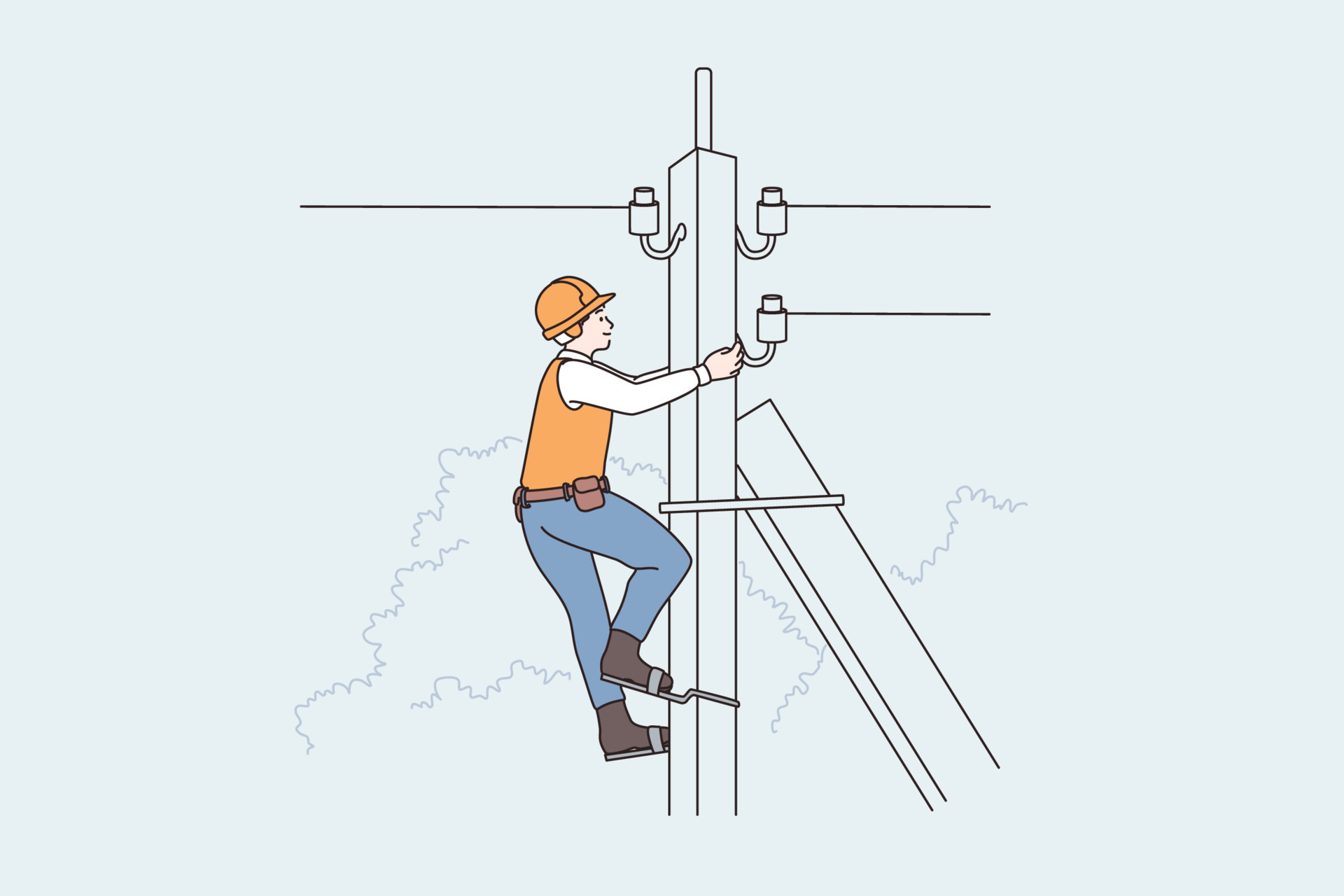The image showcases a simplistic cartoon drawing, primarily rendered in black ink on a light gray background, with focal color accents on the main character. A Caucasian lineman, characterized by his pale skin, is depicted climbing a rectangular, pole-like structure. His attire includes an orange helmet and vest, a white long-sleeve shirt, blue jeans, and black boots, along with a utility belt equipped with various attachments. Using a metal foot apparatus, the lineman ascends the pole, which has three wires extending from its top. The background is minimalistic, featuring light gray tones and faint outlines of trees, emphasizing the straightforward and basic pen-and-ink style of the illustration.